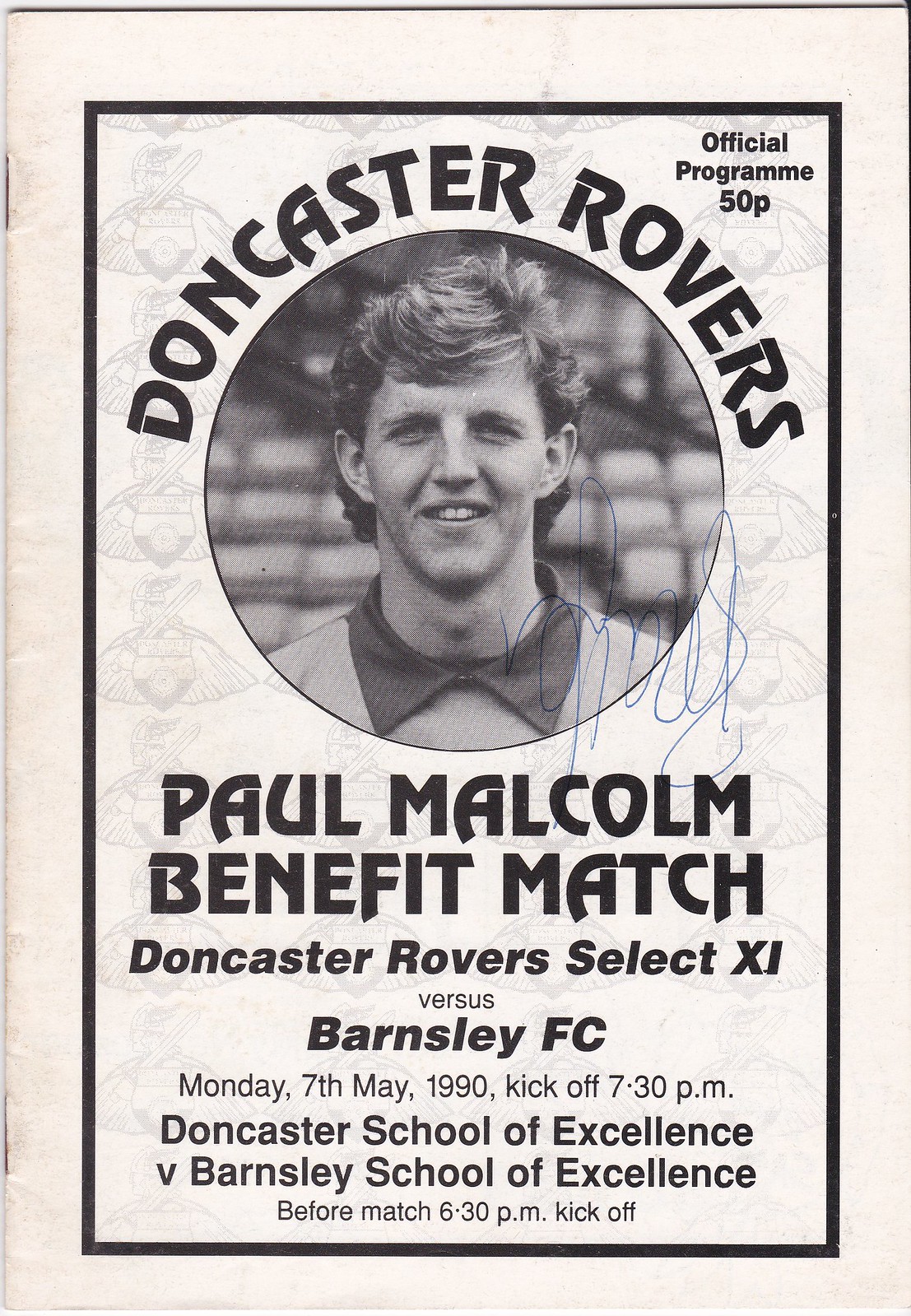The cover of the official program printed on white paper features a solid white border with an inner black line framing the content. The background within this black-bordered rectangle consists of a semi-transparent, repeating Doncaster Rovers insignia. At the top, in black text wrapping around a photograph of a young man’s face, are the words "Doncaster Rovers." The top right corner of the cover reads "Official Program 50P." Below the centrally positioned black-and-white photograph, which appears to be of a soccer player and includes an autograph on its bottom right corner, the text reads: "Paul Malcolm Benefit Match Doncaster Rovers Select XI vs. Barnsley FC. Monday 7th, May 1990, Kickoff 7.30pm." Further details include a smaller print announcement of a preliminary match: "Doncaster School of Excellence vs. Barnsley School of Excellence, before match 6.30pm, Kickoff."